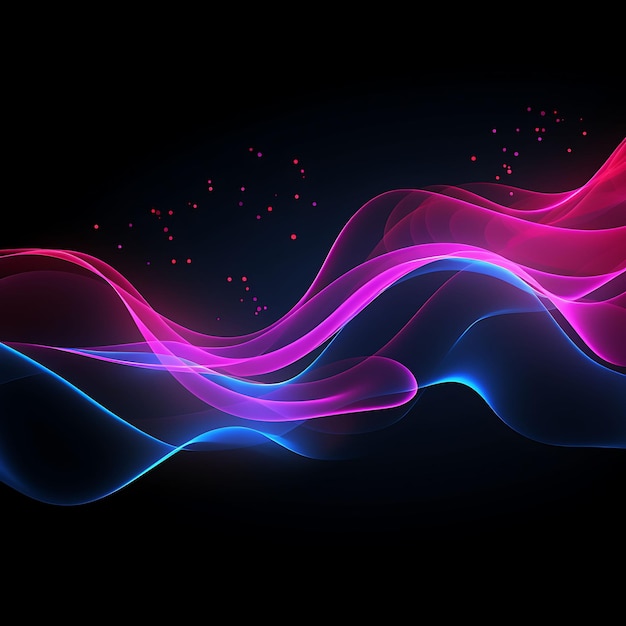This computer-generated image prominently features wavy, translucent waves of color in magentas, purples, and blues, set against a solid black background. The waves, reminiscent of smoky soundwaves, traverse from left to right, beginning thin on the left and becoming progressively thicker towards the right. The magenta and blue waves, interwoven and flowing naturally, dominate the center of the image with bright white highlights accentuating their movements. Above these vibrant waves, the upper portion of the image is speckled with numerous tiny dots in matching hues of orange, pink, and purple, adding a dynamic, ethereal quality. The dots are concentrated above the waves, leaving the lower half free of this polka dot detailing, enhancing the contrast and visual depth of the composition.